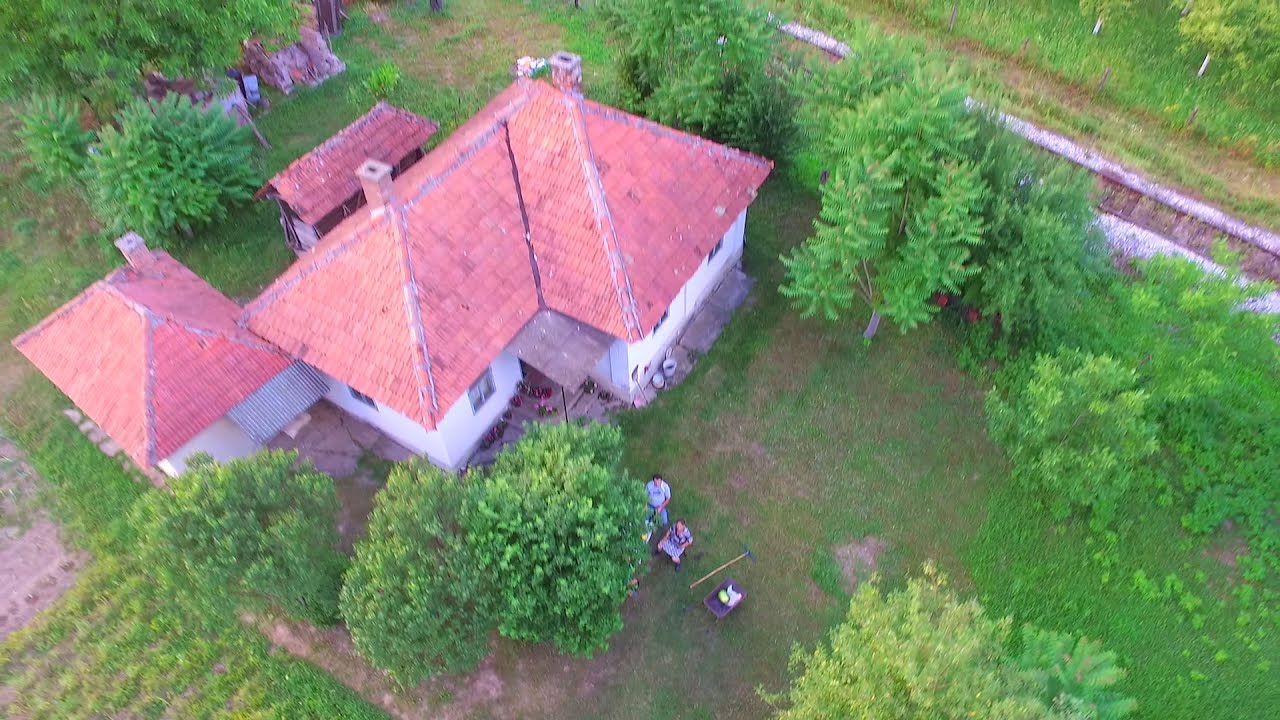This aerial photograph, likely taken by a drone, reveals a small, rectangular single-bedroom house characterized by its red brick or red tile roof and white exterior walls. The roof is adorned with three chimneys. The house is set in a lush, green yard densely populated with approximately 10 to 15 trees, suggesting a tropical location possibly in South America or Europe. Surrounding the house, there's a mixture of green grass and small garden plots. 

Adjacent to the house, on one side, stands a detached small red-roofed building, possibly a garage or shed, matching the house's roofing style. In this large yard, there are two people visible, one who might be a man and the other possibly a woman. They appear to be looking up towards the camera, with gardening instruments such as a shovel and a wheelbarrow placed nearby. The broader surrounding area appears to include some farmland, further contributing to the rural ambiance of the scene.